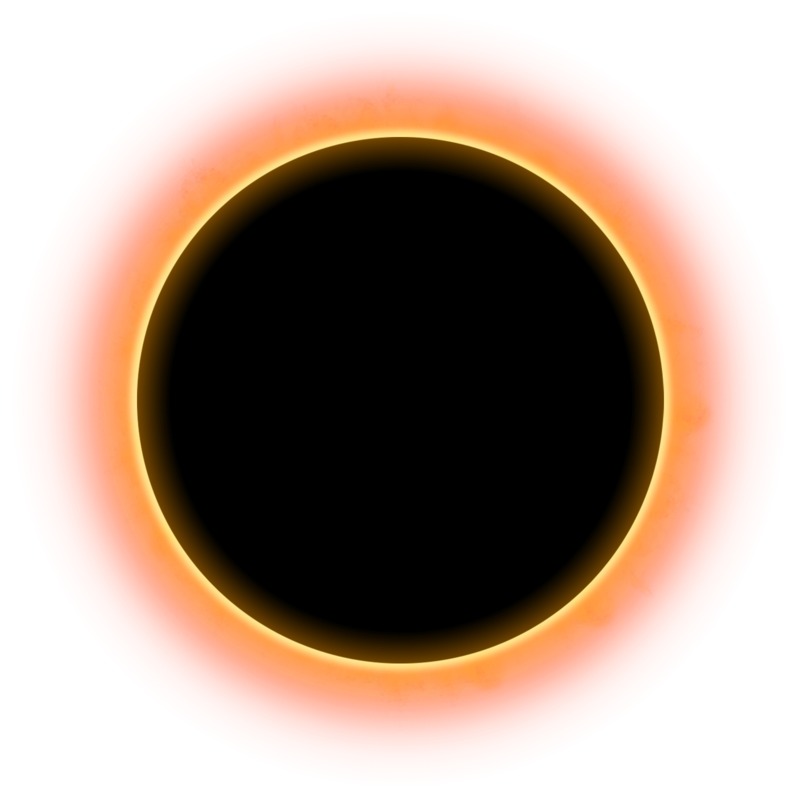The image is a detailed and artistic representation of a solar eclipse, illustrated against a white background. At the center, a solid black circle signifies the moon moving in front of the sun. The black area appears almost transparent, giving a subtle orange hue at its edges. Surrounding this, a brilliant yellow ring traces the inner edge of the eclipse, symbolizing the outer edge of the sun obscured by the moon. Radiating outwards from the yellow ring is a thicker, fuzzy orange halo, blending seamlessly into the background. The depiction vividly captures the celestial phenomenon with stark contrasts and vibrant colors, creating a resemblance to a glowing pupil encircled by an intense aura of light.